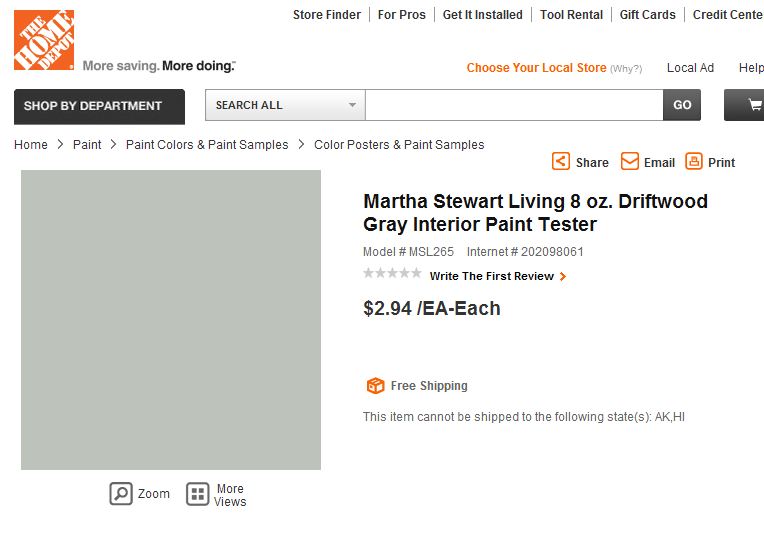A screenshot of the Home Depot website is displayed, showcasing its user interface and product offerings. At the top center of the page, various navigation options are visible, including "Store Finder," "For Pros," "Get It Installed," "Tool Rental," "Gift Cards," and "Credit Center." The Home Depot logo is located in the top left corner, accompanied by the brand's slogan, "More Saving. More Doing." Below the logo, additional links such as "Choose Your Local Store," "Local Ad," and "Help" are available.

The left-hand sidebar offers the ability to shop by department or conduct a site-wide search. Prominent navigation categories include "Home Paint," "Paint Colors and Paint Samples," and options to "Share," "Email," or "Print" the page contents. 

The main content of the page features the "Martha Stewart Living 8 oz. Driftwood Gray Interior Paint Tester," with model number MSL265 and internet number 22098061. The product is listed at a price of $2.94 each, and it currently has no reviews, inviting users to "Write the first review." Although the image of the product is not displayed, detailed product information is provided.